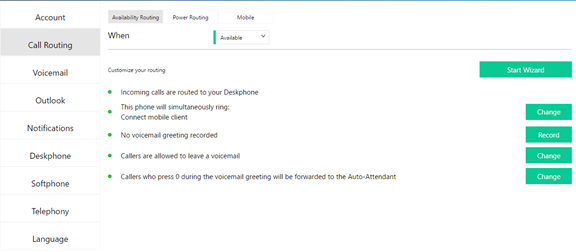This detailed caption describes a screenshot from a modern-designed website or app interface focused on call routing and telephony settings:

---

The screenshot showcases a sleek, bright-white webpage with a user interface designed for managing telephony settings. On the left side panel, there are several navigation tabs in gray, including "Account," "Call Routing," "Voicemail," "Outlook," "Notifications," "Desk Phone," "Soft Phone," "Telephony," and "Language."

The main content area prominently displays the "Call Routing" page. At the top, gray navigation tabs indicate subsections such as "Availability Routing," "Power Routing," and "Mobile." The interface features a significant text header that reads "When," accompanied by a drop-down menu currently set to "Available," highlighted with a green accent that complements the overall green theme.

Below a gray divider, the text "Customize your routing" appears next to a green button labeled "Start Wizard." Various bullet points detail customizable routing preferences:

1. Incoming calls are routed to your desk phone.
2. The desk phone will simultaneously ring a connectable client (with a "Change" button adjacent).
3. No voicemail greeting is recorded (with a "Record" button to the right).
4. Callers are allowed to leave a voicemail (with a "Change" button nearby).
5. Callers who press zero during the voicemail greeting will be forwarded to the auto attendant (another "Change" button is provided).

The user-friendly arrangement of settings and options allows for efficient customization of call routing preferences.